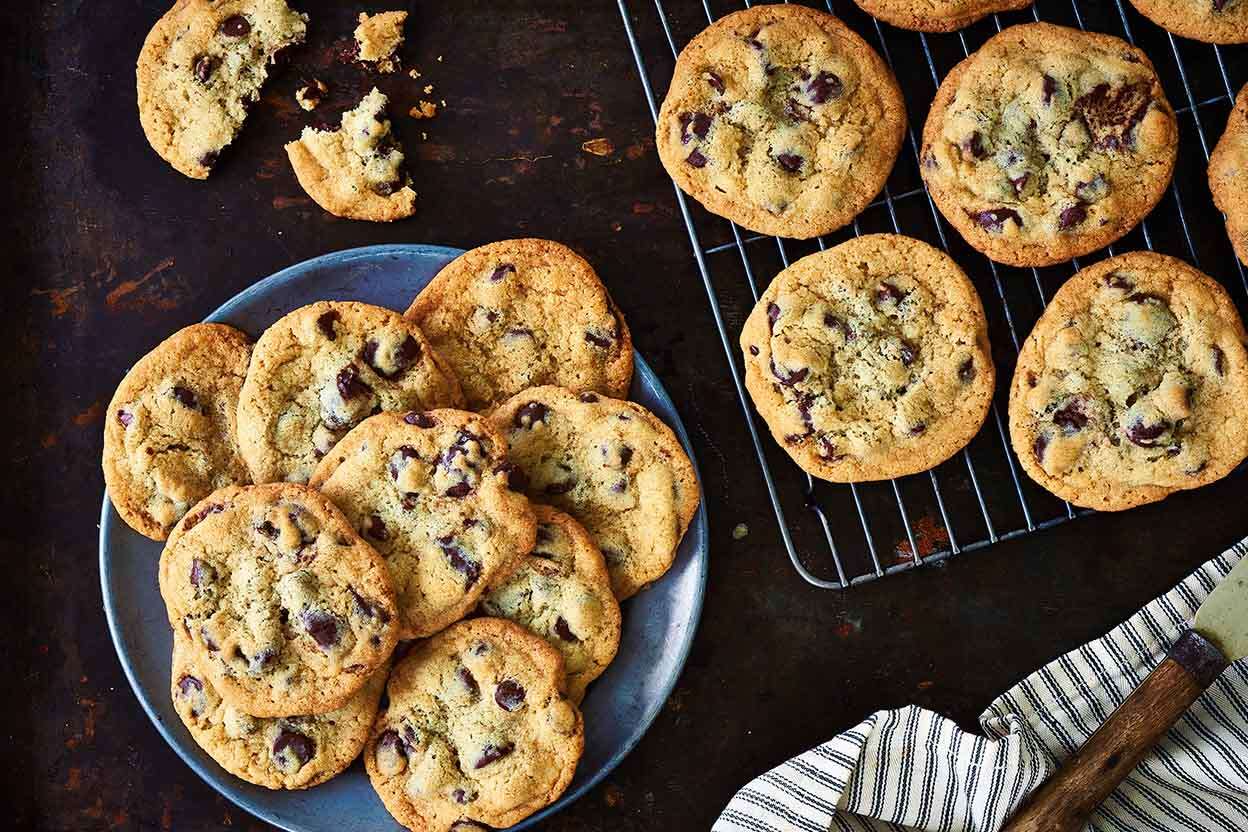This vertical rectangular photograph captures freshly baked chocolate chip cookies in a cozy kitchen setting. Dominating the bottom-left corner, a blue plate holds a generous pile of light beige cookies with neatly interspersed brown chocolate chips. Adjacent to the plate on the tabletop, there is a partially eaten cookie, crumbled with small crumbs scattered around. The dark brown table surface—though not clearly wood-grained—provides a rich contrast to the cookies. On the upper right, a metal cooling rack supports another batch of cookies, suggesting they were recently taken out of the oven. A black and white striped towel is casually draped on the counter near a wooden-handled spatula, an essential tool for transferring the treats from baking sheet to cooling rack. The overall scene conveys the warmth and delight of home baking.